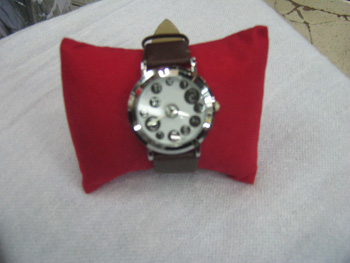A luxurious and elegant wristwatch, showcasing meticulous craftsmanship, is prominently displayed in this image. The watch is secured on a small red pillow, drawing immediate attention to its sophisticated design. The face of the watch is a pristine white, encircled by unique numeral markers that vary in size and are elegantly positioned around the edge. The watch's center is finished in a sleek silver, matching the chrome-like sheen of the watch hands and outer casing. The highly reflective, shiny appearance of the casing enhances the watch's opulent aesthetic. Complementing the elegant timepiece is its dark brown band, which appears to be made of high-quality leather, adding a touch of classic sophistication. The entire arrangement, with the red pillow resting atop a square white pillow, beautifully contrasts to highlight the exquisite details of the wristwatch.